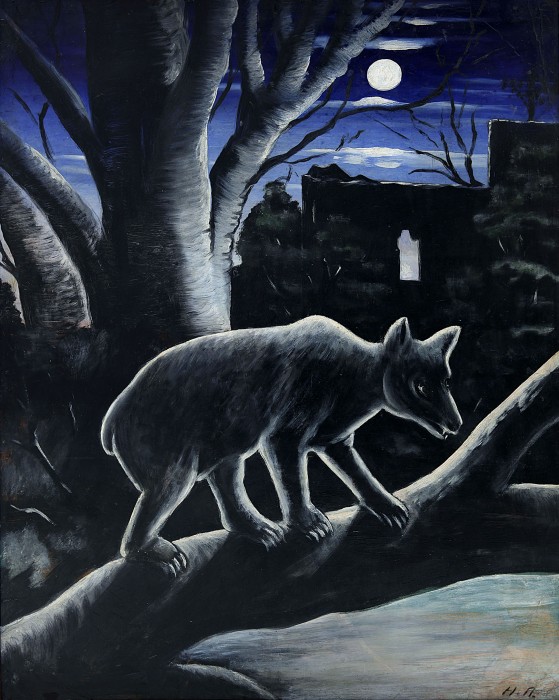The image is a detailed painting of a dark grey or black animal, possibly a wolf, coyote, or opossum, resting on a bare, low-lying tree branch that is almost parallel to the ground. The animal has short, close-to-body fur and features a sharp head with two ears, a short tail potentially curled to the left side, and is facing to the right. Its front left leg is forward, with the other three legs positioned behind. It possesses four claws on its front paws, and three claws on its back right leg. The foreground shows a nearly leafless tree, while an even larger, thicker tree looms behind the creature. In the background, a full moon illuminates the scene, casting light on the animal and the trees, and sits above a black stone wall or building, potentially with a large open window. To the top right, there are some light clouds and a body of light blue water is visible below. The drawing, which has an artist's signature at the bottom right, appears to be created with colored pencils, adding to the intricate detailing of this serene, moonlit landscape.